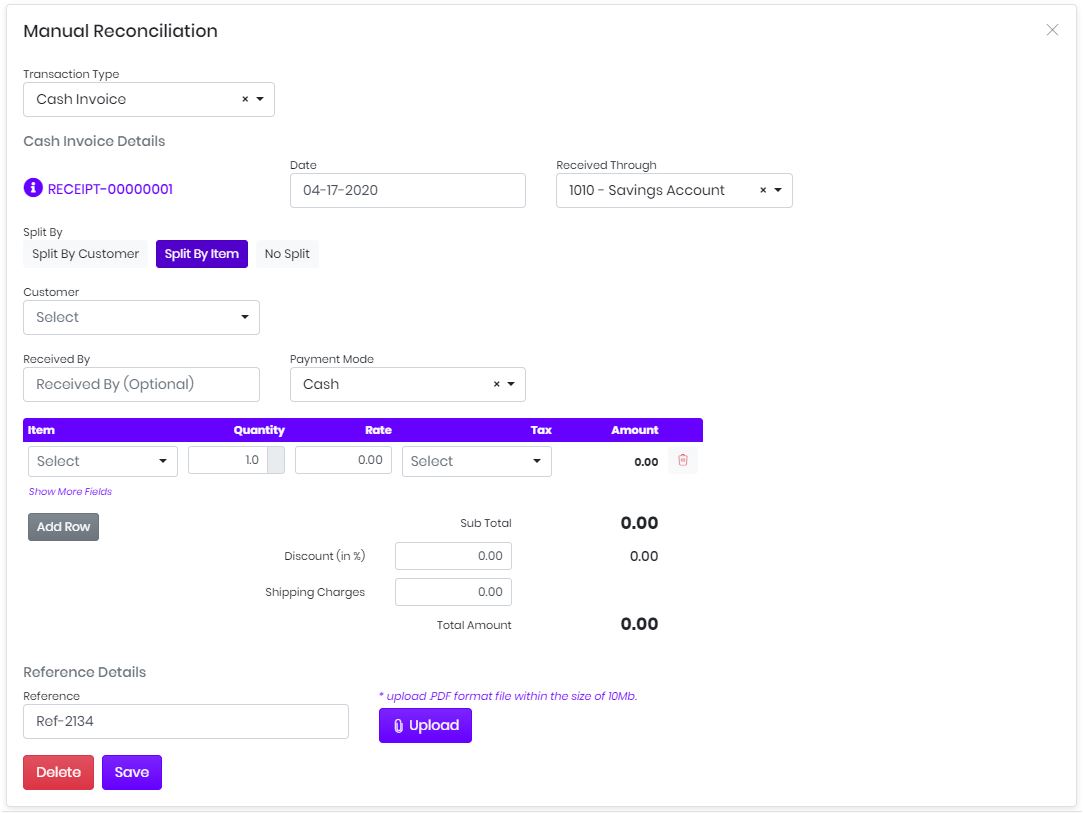**Detailed Caption:**

The image displays a white user interface screen, identified at the top left corner as "Manual Reconciliation". On the top right corner, there is an 'X' symbol which serves as an exit button for the screen. Below the title, "Manual Reconciliation," there is a field labeled "Transaction Type" with a dropdown box that currently shows "Cash Invoice." This field is accompanied by an 'X' symbol and a dropdown arrow.

Below the "Transaction Type," there is a header "Cash Invoice Details." Under this header, a purple circle with an 'i' icon is present, followed by the text "Receipt 00000001" in purple. Adjacent to this, the field "Date" shows a placeholder in the format 04-17-2020. Next to the date field is the label "Received From," coupled with a dropdown box set to "1010 - Saving Account." This field also features an 'X' symbol and a dropdown arrow.

Under the "Receipt" section, there is an option labeled "Split By," with three possible choices: "Split by Customer," "Split by Item," and "No Split." The "Split by Item" option is highlighted in purple. Beneath the "Split by Customer" option is a "Customer" dropdown box with "Select" as the placeholder text, followed by a dropdown arrow. Further below is the label "Received By," and an empty box with "Received By (optional)" inside.

Further down, there is a field for "Payment Mode" with a dropdown box containing "Cash," alongside an 'X' symbol and a dropdown arrow. Below this, a purple bar categorizes subsequent fields: Item, Quantity, Rate, Tax, and Amount. 

- The "Item" category has a dropdown box showing "Select."
- Under "Quantity" is an empty box with the number 10.
- The "Rate" box is showing 0.00.
- The "Tax" field has another dropdown box labeled "Select."
- The "Amount" displays 0.00.

A red trash can icon is present beside the "Amount" field. Under the "Item" category, a button labeled "Show More Fields" appears in purple, and below this, a grey button labeled "Add Row."

Further down, under "Quantity" and "Rate," there are additional fields labeled "Discount (%)" and "Shipping Charges." 

- The "Discount" field contains a box with 0.00.
- Adjacent to the "Shipping Charges" field, there is a box with 0.00.

Above these fields is the label "Subtotal," showing 0.00. The "Total Amount" appears below "Shipping Charges" with its value also showing 0.00.

At the bottom of the screen, there are "Reference Details," starting with a "Reference" field that showcases "ref-2134." To the right, there is a prompt in purple reading "Upload PDF format file within the size of 10 MB," accompanied by a purple button with a paperclip icon labeled "Upload." Beneath the "ref-2134" field, there are two buttons: one red button labeled "Delete" and another purple one labeled "Save."